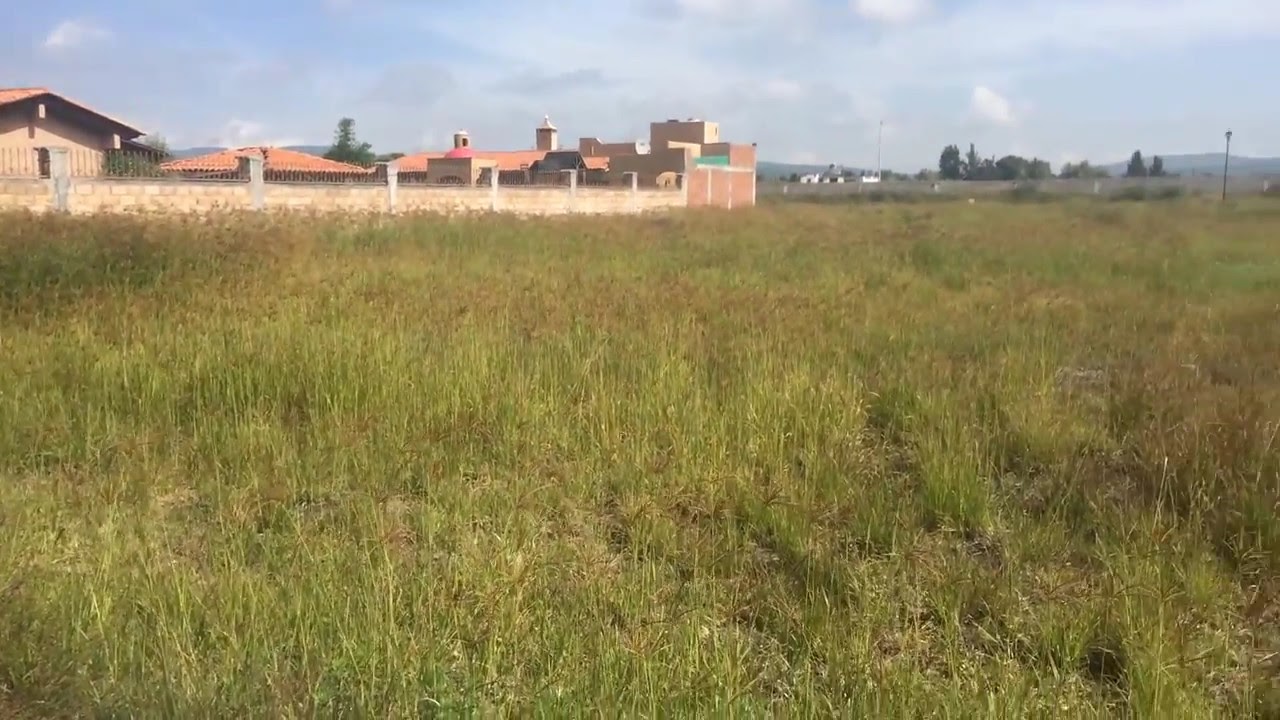The image depicts an expansive grassy meadow that occupies the majority of the frame, characterized by a mix of green and yellow grasses, along with some weeds that have brown tops. Stretching from the bottom foreground into the distance, the open field gives way to a residential area encircled by a large concrete or brick wall. This wall features gray posts and sections of fencing, possibly made of metal. Behind the wall, the residential buildings appear to be of a Middle Eastern architectural style, with light brown and beige façades, some topped with terracotta tiled roofs, and others featuring towers and domes. On the left side of the image, these buildings are interspersed with trees and occasional white structures. In the far background, a series of hills and a blue-hued mountain range can be seen under a partly cloudy, light blue sky. The entire setting suggests a daytime scene, devoid of any people, emphasizing the serene, game-like quality of the landscape.